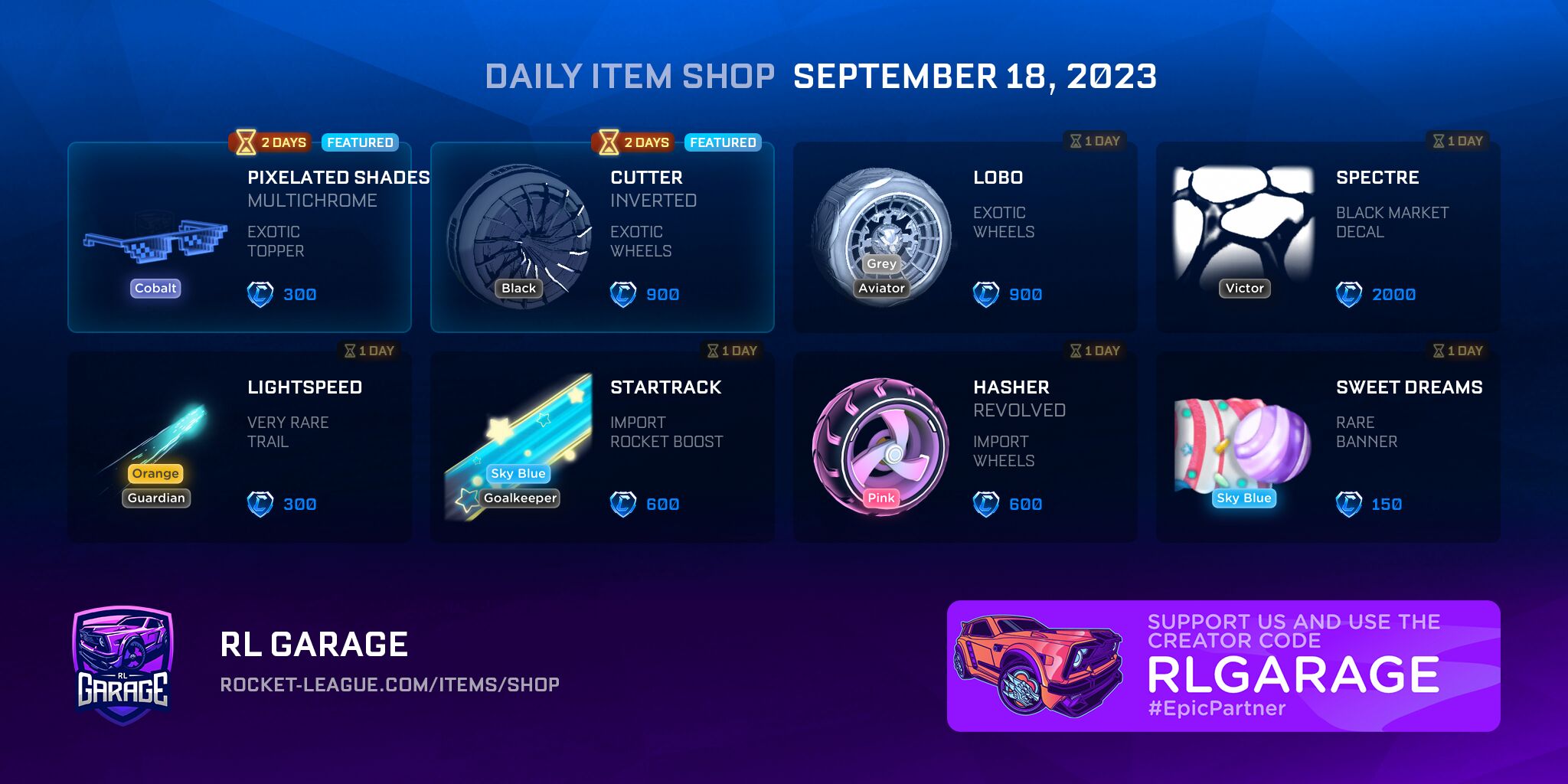Here's a detailed and cleaned-up caption for the image:

---

This post displays a detailed menu for the "Daily Item Shop" dated September 18, 2023, featuring various items available for purchase. The highlighted items include "Picolated Shades," "Boutique Chrome," an "Exotic Topper," and "Cutter Inverted Exotic Wheels." Additionally, the menu lists other non-featured items, which encompass a wide range from wheels and black market decals to banners and rocket boost trails, all for the popular game Rocket League.

In the bottom left corner, the image directs users to visit RLGarageRocketLeague.com/item/shop for more information. Meanwhile, the bottom right corner encourages support by using the creator code 'RLGarage' with the hashtag #EpicPartner. Accompanying this is a logo featuring a red car adorned with detailed flaming designs on the front.

The menu's design features a light-colored top portion transitioning to a more purple hue at the bottom, providing a visually appealing contrast and drawing attention to the different sections of items.

It appears that this shop is being promoted to gather funds for future projects, marked strategically to attract Rocket League enthusiasts.

---